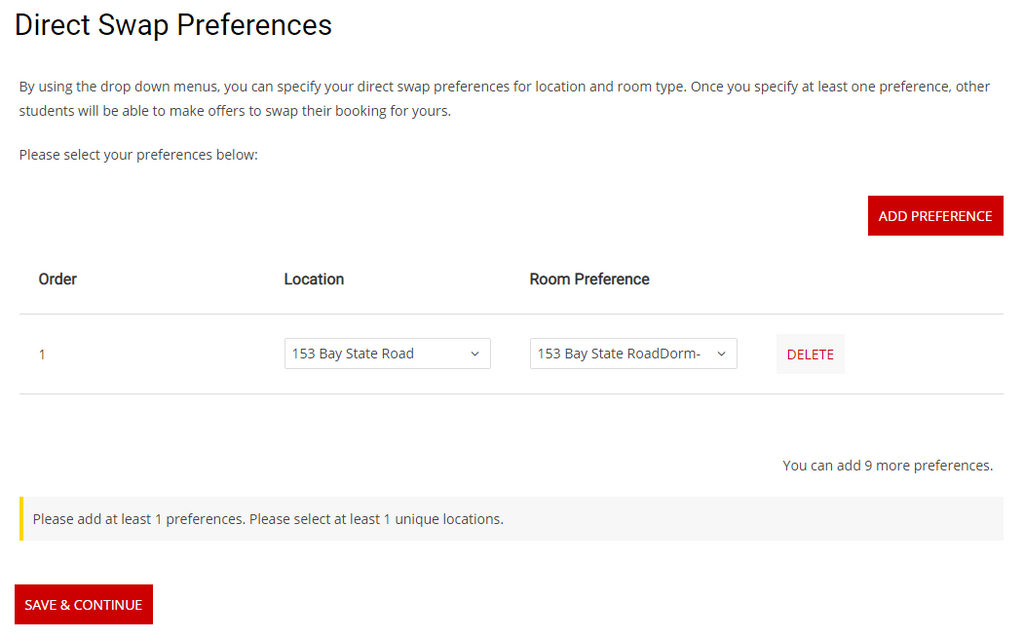The screenshot showcases a user interface with a predominantly white background, designed for specifying direct swap preferences. It includes a series of dropdown menus allowing users to select their desired criteria for location and room type. When at least one preference is chosen, other students can propose a booking swap.

Highlighted features:
- The prominent red rectangle button labeled "Add Preference" enables users to input new preferences.
- A detail entry, labeled as "Order 1," specifies a location at "153 Bay State Road" under both "Location" and "Room Preference" categories.
- A gray rectangle next to the entry contains a red "Delete" button for removing the preference.
- A note indicates that users can add up to nine more preferences.
- A gray message box prompts users to add at least one preference and select at least one unique location.
- A final red rectangle button labeled “Save and Continue” allows users to finalize their preferences.

This setup provides an intuitive and detailed method for managing room swaps, ensuring clear communication and streamlined functionality.